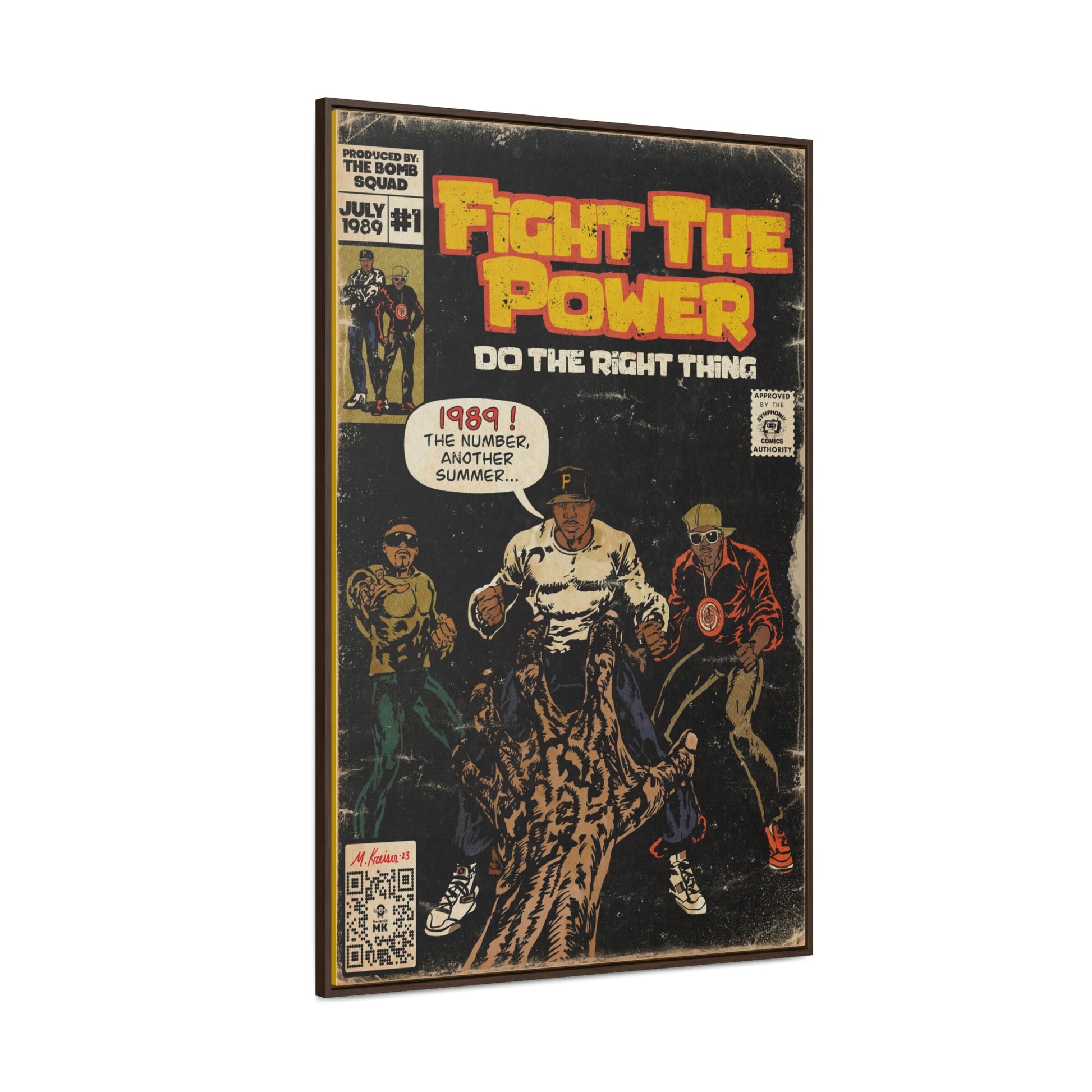The image is a photograph of a comic book cover titled "Fight the Power: Do the Right Thing." Dominating the center are three men depicted in a dynamic, comic book style. The first man on the left is an African-American wearing a Pittsburgh Pirates baseball cap and white clothing. A hand is reaching out toward him, and he has a speech bubble that reads, "1989 the number, another summer." To his right is another man adorned in a red and green tracksuit with a backward baseball cap. To the far left stands a man wearing sunglasses and a yellow and blue suit.

The top of the comic book prominently features the text "Produced by The Bomb Squad, July 1989, Number One," along with the main title. Below, two smaller superheroes are also illustrated, contributing additional intrigue to the cover's vibrant narrative. At the bottom of the comic book, there is a QR code, indicating it is likely a modern reprint or recent version.

Overall, the cover merges nostalgic visual elements with modern touches, creating a striking and culturally resonant piece.